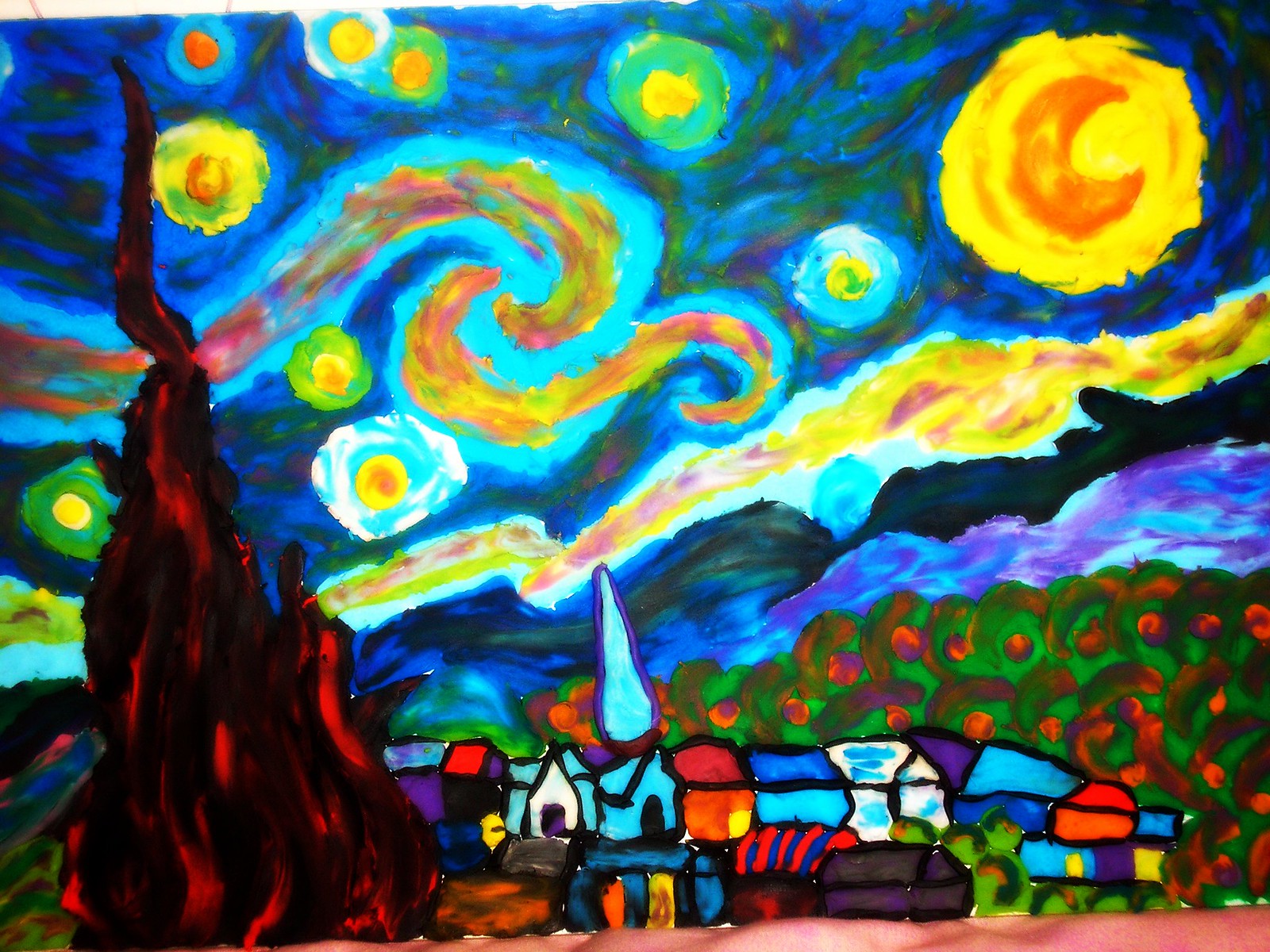The image depicts a unique rendition of Vincent van Gogh's famous painting, "Starry Night." This reimagined version features a sky composed of various shades of black, green, and blue, creating a rich and enveloping night sky. Distinctive, colorful round orbs in hues of blue, yellow, red, and green represent the stars, punctuated by swirling patterns. In the upper right corner, an orange crescent shape inside a yellow circle symbolizes the moon, adding a striking focal point.

The lower portion of the image includes a landscape that resembles a town painted with bright, vivid colors, suggesting a surrealistic townscape with a stained glass or puffy paint texture. On the left, a striking black and red form rises upwards, resembling a pointed mountain or a flame, contrasted against the subdued background. The right side features foliage that looks like green and orange bushes or a hedge with red apples, imparting an organic texture to the scene.

Overall, the artwork diverges from Van Gogh's original style with its bold use of color and shape. The color palette extends to the lower half with a variety of tones, including tones of blue and accents of purple water. The sky displays greater complexity with swirling greens and light blue highlights, creating a beautiful yet unconventional reinterpretation of the iconic masterpiece.